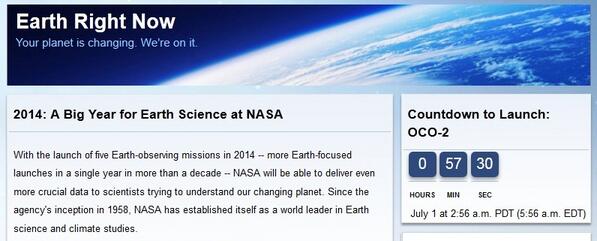The image features a gradient background transitioning from dark blue at the top to a lighter blue and eventually to white towards the bottom. The horizon of Earth as seen from space is visible at the lower edge of the frame. In the upper left-hand corner, there are white letters that read "Earth Right Now," with smaller blue letters below that stating, "Your planet is changing. We are on it."

Beneath this text, there is a white bar with the message: "2014, a big year for Earth science at NASA." It continues with, "With the launch of five Earth observing missions in 2014, more Earth-focused launches in a single year in more than a decade. NASA will be able to deliver even more crucial data to scientists trying to understand our changing planet. Since the agency's inception in 1958, NASA has established itself as a world leader in Earth science and climate studies."

Adjacent to this bar is a smaller, separate white box. The top half of this box contains black letters displaying a countdown: "Countdown to launch OCO-2: 0 hours, 57 minutes, 30 seconds." It specifies the launch time as "July 1st at 2:56 a.m. Pacific Time, 5:56 a.m. Eastern Time."